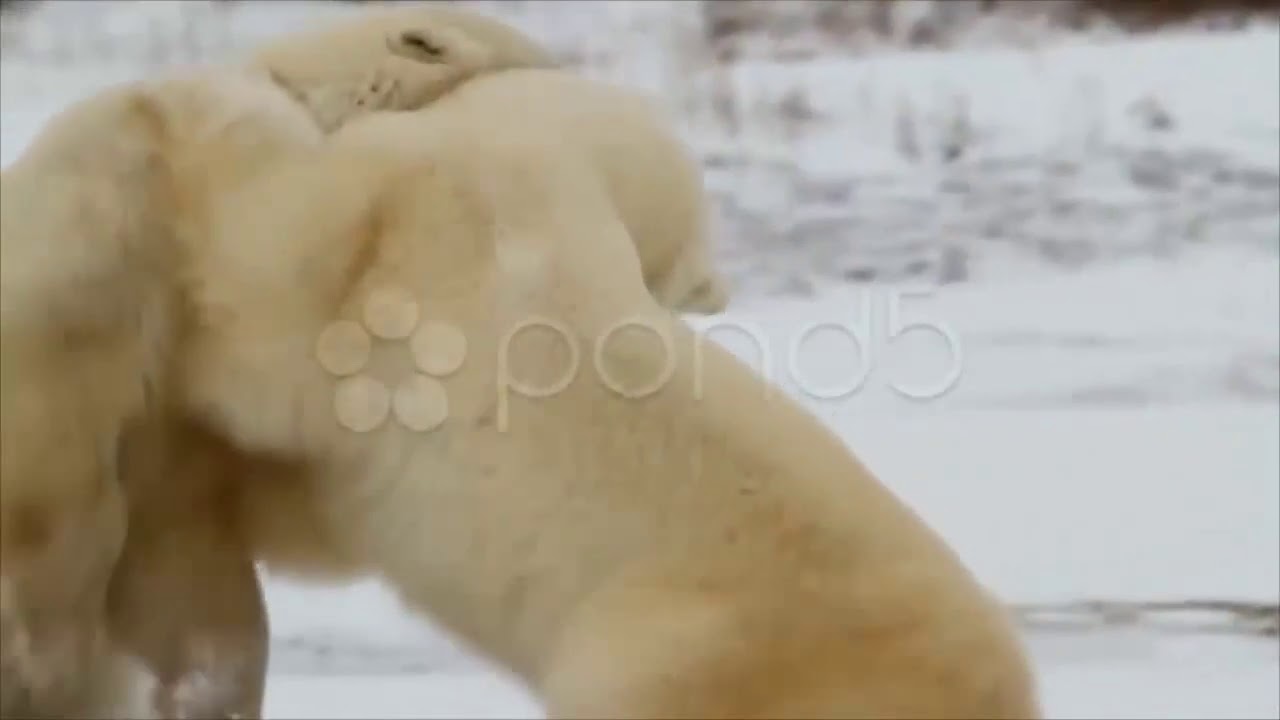The image depicts a snowy winter scene featuring two light-colored animals, either polar bears or panda bears, standing on their hind legs in the foreground. They appear to be interacting playfully, as one animal embraces the other from behind in what resembles a wrestling or hugging pose. Their heads are turned away from the camera, making it difficult to see their faces clearly. The animals have an off-white or yellowish-white coloration, possibly with some brown patches. The background is blurred, emphasizing the snowy ground with occasional bumps and a jagged, brownish area in the upper right corner that might be rocks or vegetation. A watermark resembling a flower with five petal-like circles and the text "Pond5" is prominently placed in the center of the image.